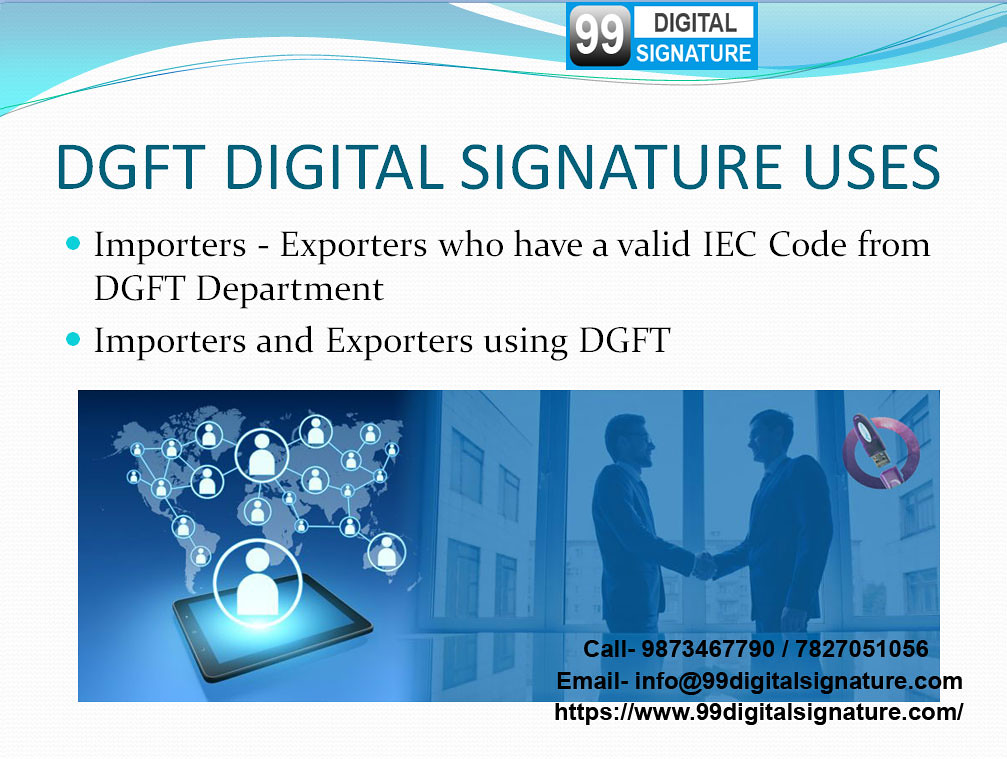The image is a detailed promotional slide for "99 Digital Signatures," specifically focusing on the uses of DGFT Digital Signatures. At the top right, the text prominently displays "99 Digital Signature" in large teal font, followed by "DGFT Digital Signatures Uses." Below this, bullet points highlight that importers and exporters with a valid IEC code from the DGFT Department are the primary users. Another bullet point reiterates the usage by importers and exporters utilizing DGFT.

Central to the slide is a photograph with a blue tint, depicting two men shaking hands, symbolizing a business agreement facilitated by the digital signatures. To the left of this image, there appears to be a black iPad with interconnected circles above it, suggesting digital connectivity and integration.

In the lower right corner of the slide, contact information is clearly provided: phone numbers (987-346-7790 and 782-705-1056), an email address (info@99signatures.com), and the website (www.99signatures.com). The slide is designed to attract businesses to explore and adopt 99 Digital Signatures for their DGFT-related needs, encouraging them to reach out via call, email, or by visiting the website for more information.